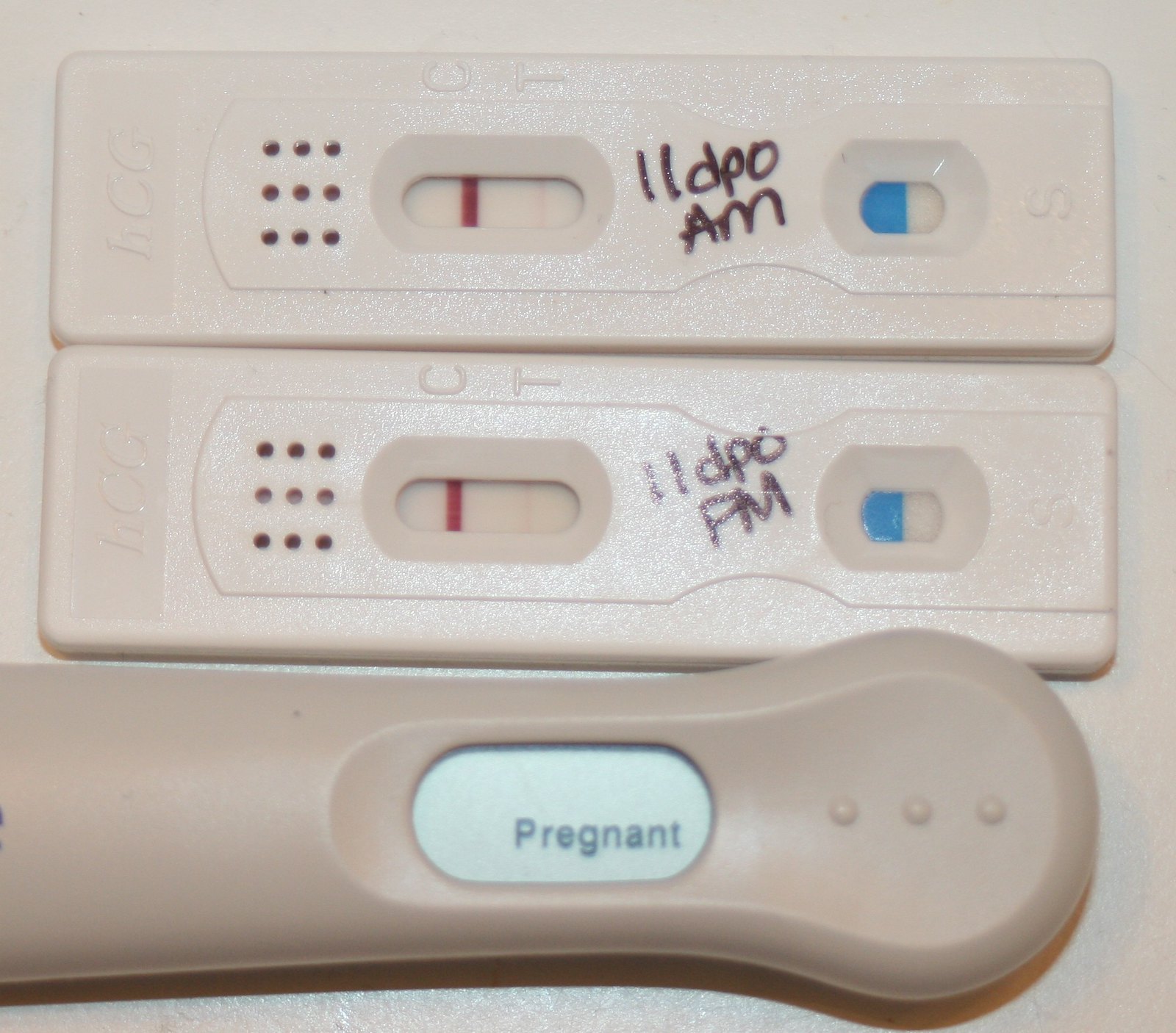The image displays three pregnancy tests positioned on a white countertop. Two of the tests appear to be from the same brand and model, while the third test is from a different brand. The top two tests have handwritten labels: "11 DPO AM" and "11 DPO PM," indicating they were taken at different times of the day on the 11th day past ovulation. These tests feature nine small dots on the left side, the purpose of which is unclear. Each of these tests has an oval window marked with a 'C' and a 'T,' suggesting a control and test indicator rather than temperature. The red indicator dot is located under the 'C' in the first window, while a blue mark is partially visible in the second window.

The third test below these two is distinctly different in design. It is more curved and has three small dots on its right side. This test has a digital display reading "Pregnant," clearly indicating a positive result. The variety in test designs and labels provides a comparative view of multiple testing instances within the same time frame.